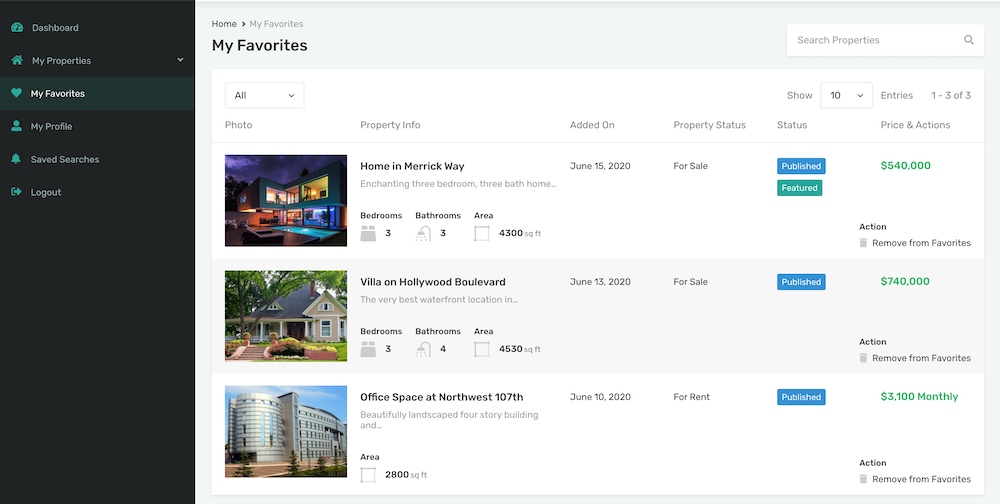Here is a detailed and cleaned-up caption for the image:

---

The image showcases a user's profile page, focusing on the "My Favorites" section. On the left side, in dark teal green, are several clickable options listed vertically: Dashboard, My Properties (with a drop-down menu), My Favorites, My Profile, Saved Searches, and Log Out.

The right side of the screen features tabs labeled "Home," "Favorites," and is currently displaying the "My Favorites" tab. In this tab, users can search for properties and view their saved favorites. Presently, three properties are listed:

1. **Merrick Way Home**: An enchanting 3-bedroom, 3-bathroom home spanning 4,300 square feet. This property, added on June 15, 2020, is for sale and listed as published and featured, priced at $540,000. An option to remove it from favorites is available.
   
2. **Villa on Hollywood Boulevard**: The very best waterfront location, featuring 3 bedrooms and 4 baths with a total area of 4,530 square feet. This listing, added on June 13, 2020, is also for sale, published, and priced at $740,000. An option to remove it from favorites is provided.

3. **Office Space at Northwest 107th**: A beautifully landscaped four-story building offering 2,800 square feet of office space, added on June 10, 2020. This property is available for rent at $3,100 per month and the status indicates published. Similarly, there is an option to remove it from favorites.

Each listing includes a photo, detailed property information, the date added, property status, publication status, and associated actions.

---